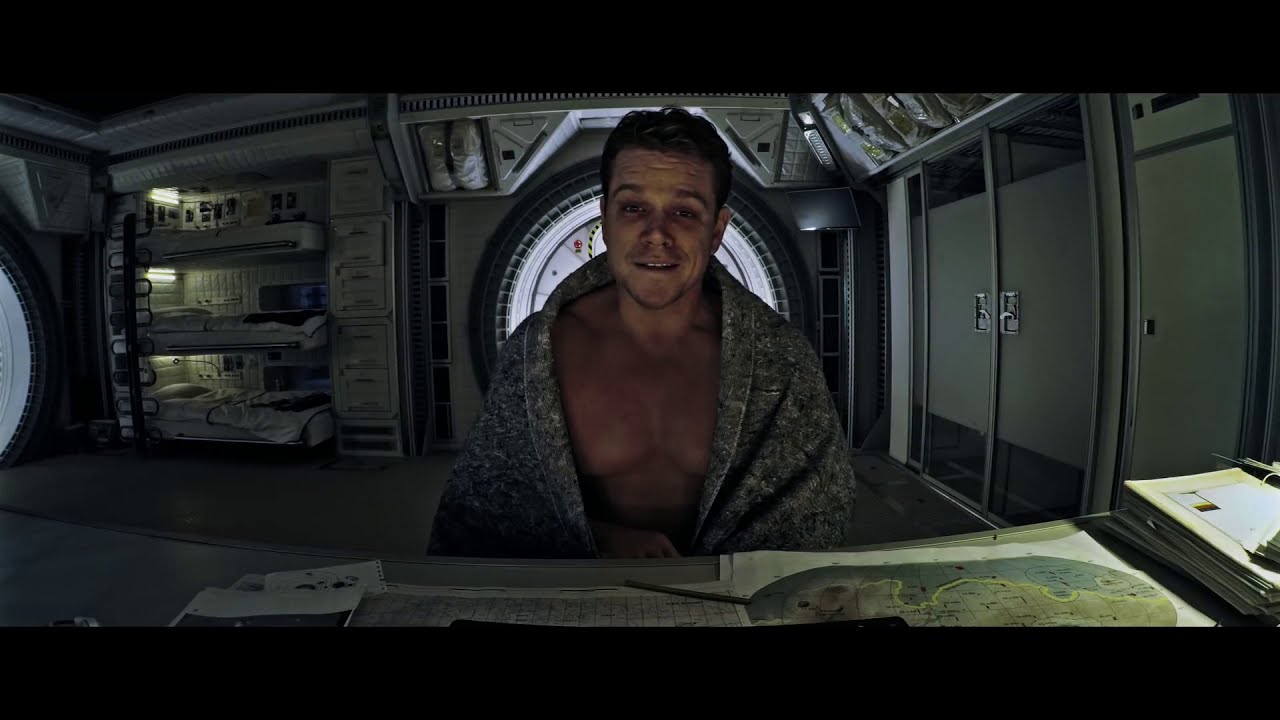The image depicts a shirtless man, his upper body wrapped in a robe speckled with black and white, sitting centrally at a desk covered with maps, documents, and a pen. He has short, slightly wavy brownish-blonde hair with a bit of scruff above his lips and faint wrinkles on his forehead. His mouth is slightly open, revealing his top teeth in a half-smile, and his muscular chest is prominently bulging outward. The room appears to be part of a spaceship, possibly from a scene in the movie "The Martian" starring Matt Damon, based on the man's resemblance to the actor. Behind him to the right, there are metal doors, likely airlocks, and to the left, three bunk beds with white cabinets. The background also features a large circular window, enhancing the futuristic ambiance. The image is framed by black borders at the top and bottom, suggesting it might be a widescreen capture from a digital screen.